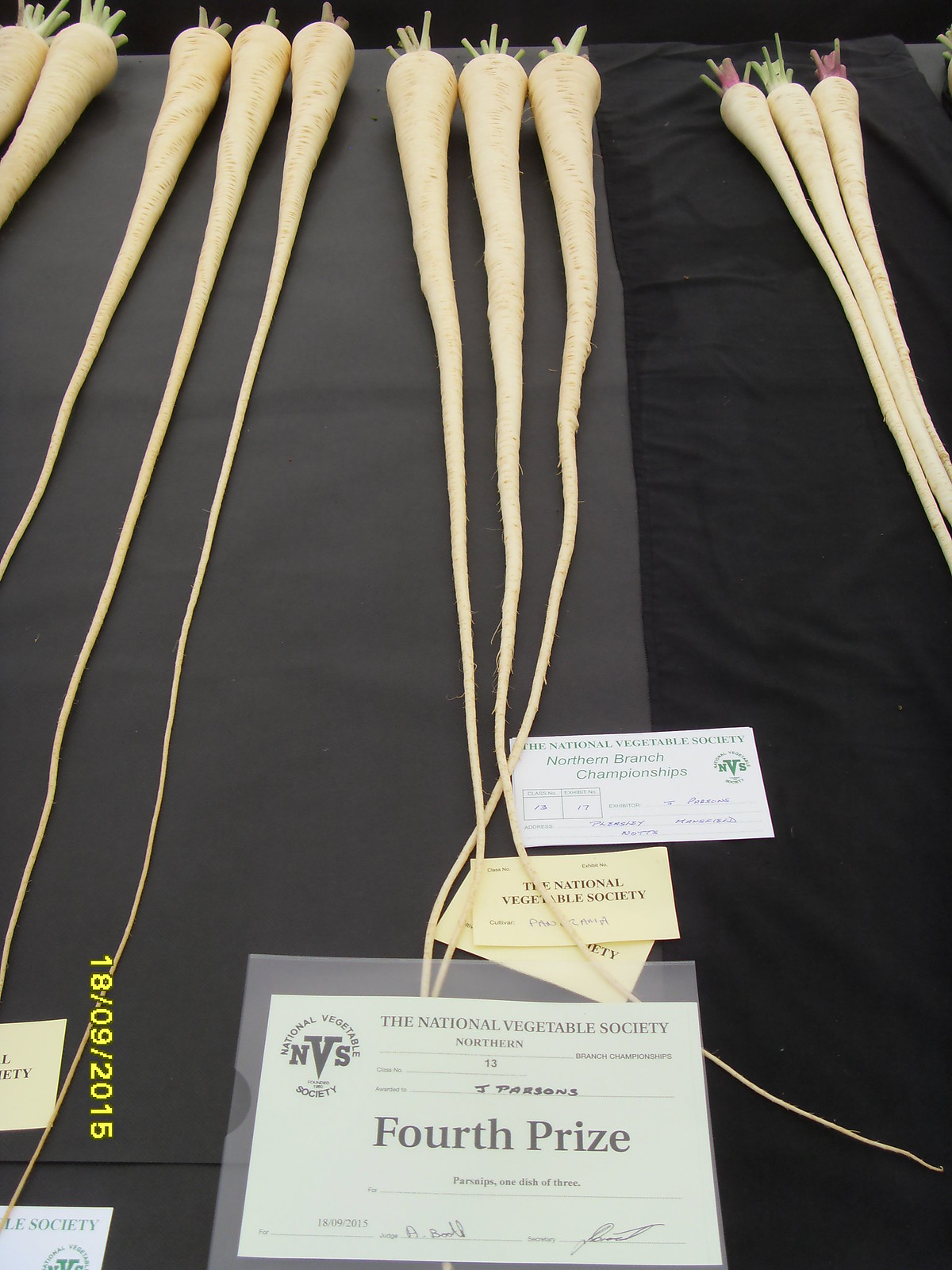This display, featured at the National Vegetable Society Northern Branch Championships, showcases a collection of long, slender parsnips with light orange to whitish-yellow coloring. These parsnips, displayed against a black and gray tablecloth, have green stems at the top tapering down to delicate roots. Notably, a white card indicates that Jay Parsons earned fourth prize for "parsnips one dish of three" in class number 13. This achievement is further corroborated by a laminated sheet and a business card beside the parsnips, both bearing the National Vegetable Society's logo and the "NVS" acronym. Each card is signed by a judge, dated September 18, 2015, adding a formal recognition to the display.